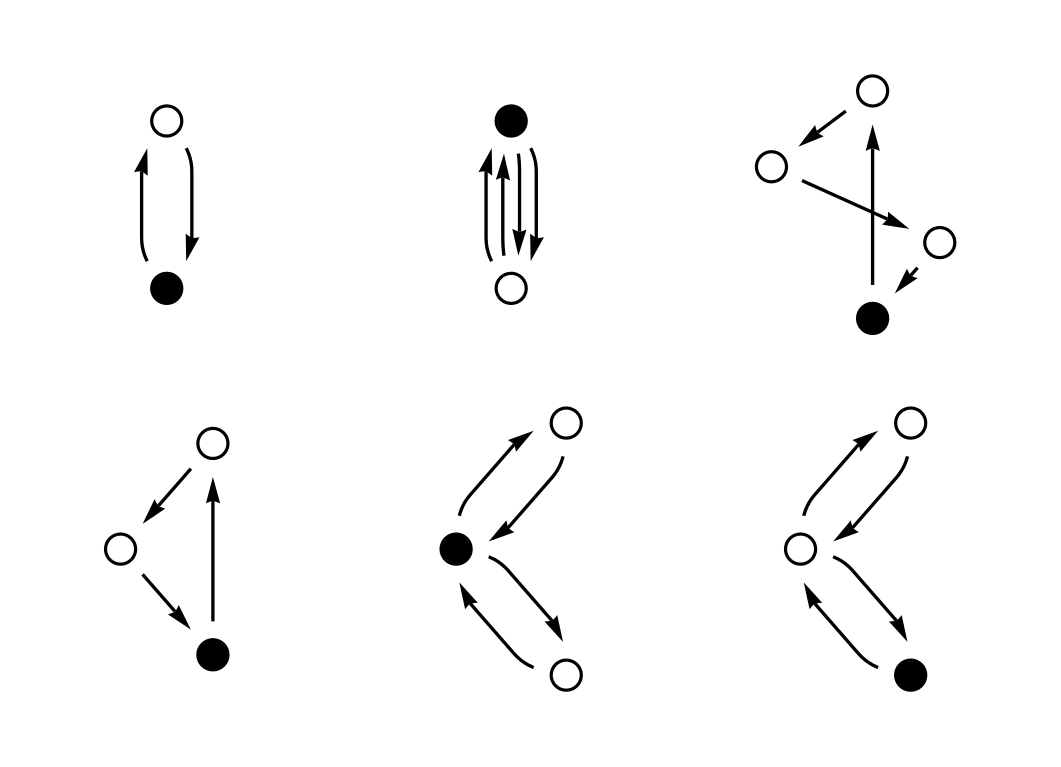The image showcases a collection of six distinct puzzles typically found in a mathematics course, neatly arranged in two rows of three. Each puzzle features a set of circles and directional arrows, creating intricate patterns. Here’s a detailed description of each:

1. **First Puzzle (Top-Left)**: It includes a white circle at the top and a black circle at the bottom. Arrows indicate a bidirectional relationship, with one arrow pointing upward from the black circle to the white circle, and another arrow pointing downward from the white circle to the black circle.

2. **Second Puzzle (Top-Middle)**: This puzzle reverses the positions, having a black circle at the top and a white circle at the bottom. Two arrows are pointing upward from the white circle to the black circle, and two arrows are pointing downward from the black circle to the white circle, suggesting a stronger emphasis on the directionality compared to the first puzzle.

3. **Third Puzzle (Top-Right)**: This features three white circles alongside one black circle. There's a complex arrangement of arrows: one arrow goes from the black circle straight up to the nearest white circle. From this white circle, an arrow points leftward to another white circle, which is connected by another arrow moving to the right and down to the third white circle. Finally, an arrow loops back from this last white circle to the black circle, creating a continuous path.

4. **Fourth Puzzle (Bottom-Left)**: Shaped like a triangle, it comprises two white circles at the upper corners and a black circle at the bottom vertex. Arrows form a loop: one goes from the top-left white circle to the top-right white circle, another from the top-right white circle to the black circle at the bottom, and a third arrow from the black circle back up to the top-left white circle.

5. **Fifth Puzzle (Bottom-Middle)**: This setup consists of two white circles and one black circle located within a triangular layout. Each pair of white and black circles is connected by bidirectional arrows, indicating a mutual relationship among all circles.

6. **Sixth Puzzle (Bottom-Right)**: Arranged in a vertical line with the white circle at the center, it includes two white circles and one black circle. The white circles are interconnected with bidirectional arrows. Additionally, there are arrows connecting the black circle with the central white circle, forming a bidirectional connection, which establishes a network of relationships between all circles.

This detailed analysis highlights both the structural similarities and the unique characteristics of each puzzle, revealing intricate patterns that challenge the solver's understanding of mathematical relationships.